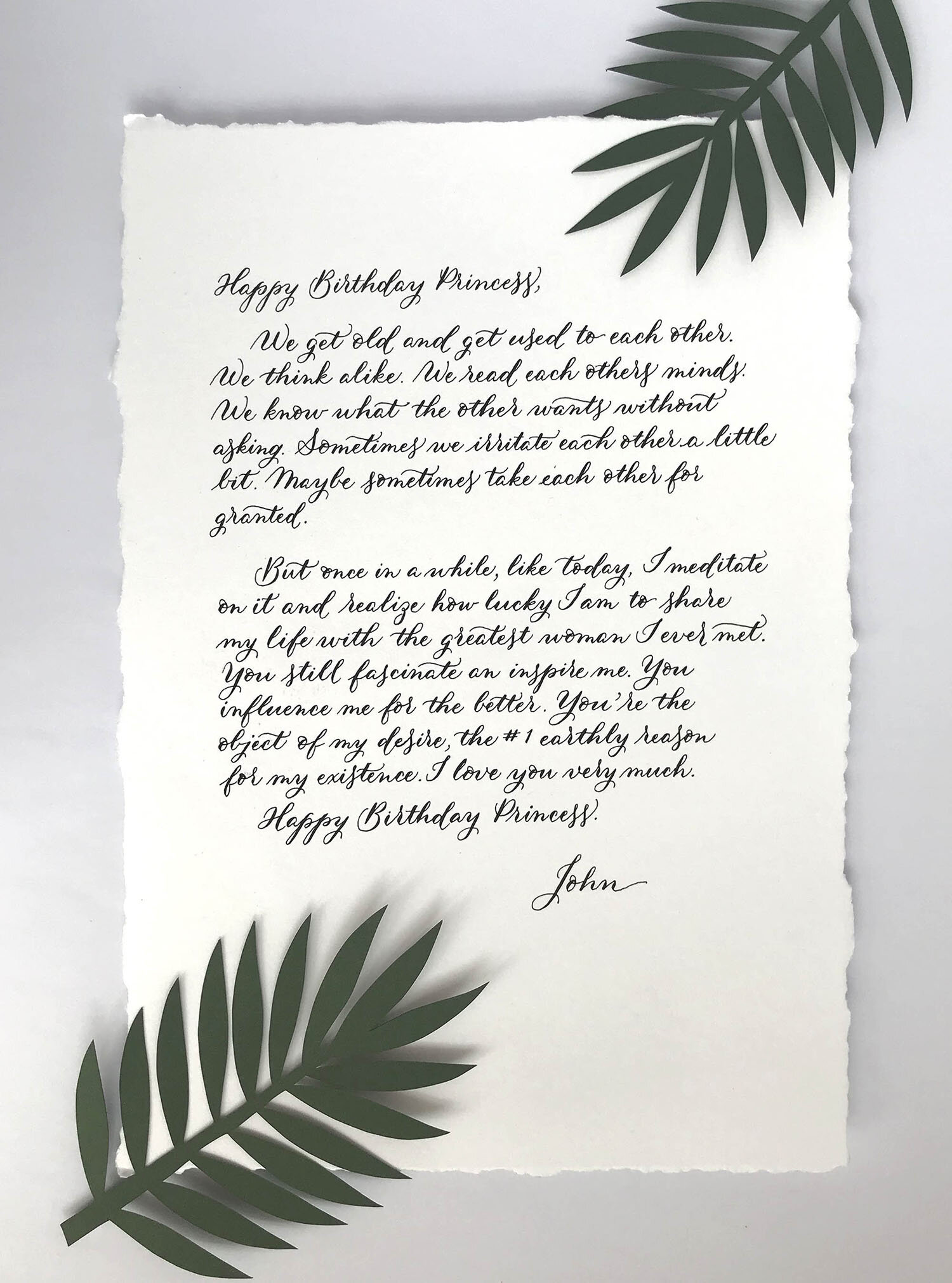The image features an unlined, white sheet of paper that appears to be torn from a notebook, with perforated edges on all sides. The paper lays flat against a light gray background. In the top right corner and bottom left corner of the image are green fern-like leaves with thin, elongated foliage, which seem to face each other. The letter on the sheet is written in a black, cursive calligraphy font and is addressed to a woman. It reads:

"Happy Birthday, Princess. We got old and got used to each other. We think alike. We read each other's minds. We know what the other wants without asking. Sometimes we irritate each other a little, and maybe sometimes take each other for granted. But once in a while, like today, I remember, I meditate on it and realize how lucky I am to share my life with you, the greatest woman I have ever met. You still fascinate and inspire me. You influence me for the better. You are the object of my desire.

Happy Birthday, Princess.
John."